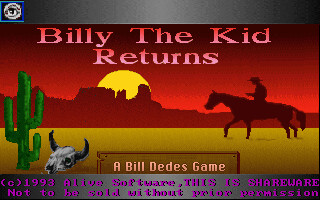This detailed and descriptive caption could be:

"The image captures the title screen of a classic arcade or video game called 'Billy the Kid Returns.' The gradient background transitions from a deep, dark red at the top to a lighter pink at the bottom, creating an ombre effect. Dominating the center of the screen, the game title 'Billy the Kid' is prominently displayed in a bold font, with 'Returns' positioned just below it. The backdrop is a dark red sky with the setting sun casting its final rays behind a rugged canyon outline. On the right side, the silhouette of a man wearing a hat rides a horse, evoking a sense of wild western adventure. The left side features a distinctive cactus next to the skull of a cow or bull. At the bottom of the screen, purple text reads 'A Bill Did His Game, copyright 1993, a live software. This is shareware, not to be sold without prior permission.' This title screen sets the tone with its atmospheric design and nostalgic elements, inviting players into the game's world."